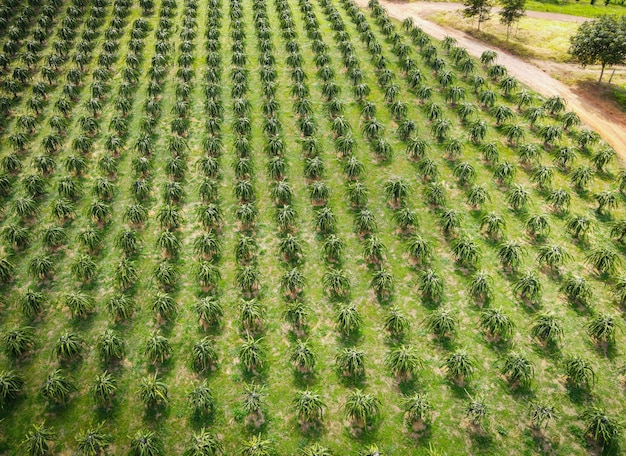This aerial image captures a vast, luxuriant green field of uniformly planted crops, meticulously arranged in perfect rows and columns. The plants, suspected to be pineapples due to their long, downward-falling leaves and frond-like appearance, cover the entire left side and central portion of the image. Throughout the field, patches of low-lying grass and bare soil can be seen, with a notable gap where one plant is missing in the center-right. On the right side of the image, a dirt road borders the field. This road has multiple turnoffs and is flanked by tall trees and additional grass. The positioning of the shadows suggests the photo was taken with the sun high in the sky. The entire scene is viewed from an elevated perspective, likely captured by a drone.